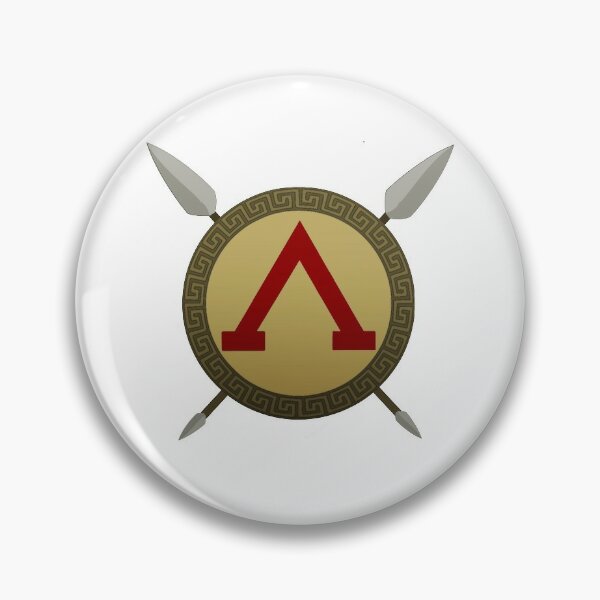The image features a minimalistic digital illustration of an ancient Greek-themed shield set against a plain white background. At the center of the composition is an off-white, lightly reflective circle featuring a detailed shield. This shield showcases a dark brown and mustard gold labyrinthine pattern along the edges, which is typical of Greek art. The central part of the shield is a light tan color and prominently displays a red upside-down V symbol. Adding to the historical theme, the shield is flanked by four spears: two large silver spears at the top left and top right, as well as two smaller spears jutting out from the bottom left and right. The overall design has a simple, yet detailed aesthetic, evocative of classical Greek armor, complete with strategically placed highlights indicating the light source from the left side of the image.